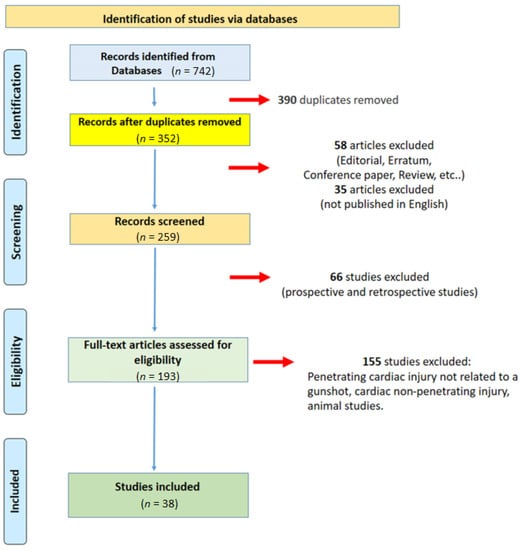This detailed flowchart, set against a white background and featuring vertical columns, visually represents the process of identifying studies via databases. At the top, within a beige box, black text states "Identification of studies via databases." Below this, a sequence of color-coded boxes outlines each step: a blue box for "Records identified from databases (N=742)," leading to a yellow box for "Records after duplicates removed (N=352)" indicating "390 duplicates removed." Following the yellow box is another blue box for "Records screened (N=259)," and a green box for "Full-text articles assessed for eligibility (N=193)" illustrating "58 articles excluded." The sequence continues with another green box for "Studies included (N=38)", alongside annotations marking "66 studies excluded" and "155 studies excluded." On the left side of the chart, four vertical blue boxes in sequence read "Identification," "Screening," "Eligibility," and "Included," each connected by red arrows to corresponding stages in the process. Additional red arrows detail exclusions, such as for "Penetrating cardiac injury not related to a gunshot, cardiac non-penetrating injury, and animal studies." The chart employs various colors (light blue, yellow, peach, off-white, and green) to enhance clarity and distinction among categories.